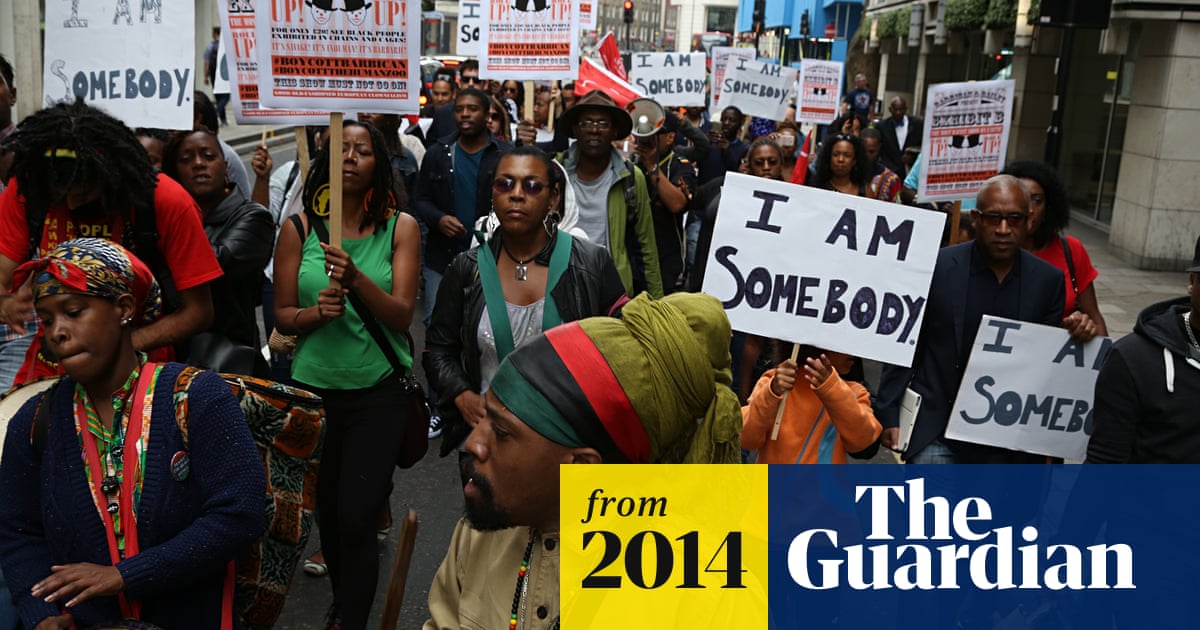The image depicts a 2014 protest on a city street, as captured in a professional photograph likely used by The Guardian, evidenced by the "From 2014" and "The Guardian" labels in yellow and navy blue in the bottom corner. The scene is filled with African-American men, women, and children, many adorned in elaborate head wraps and matching outfits. The protesters are carrying numerous signs, the most prominent of which read "I am somebody." A child is also seen holding one of these signs. One individual stands out with a megaphone. The urban setting is flanked by buildings on either side, and the sky is visible in the background, suggesting the city's somewhat narrow streets. The details emphasize the unity and determination of the protesters captured in this moment.